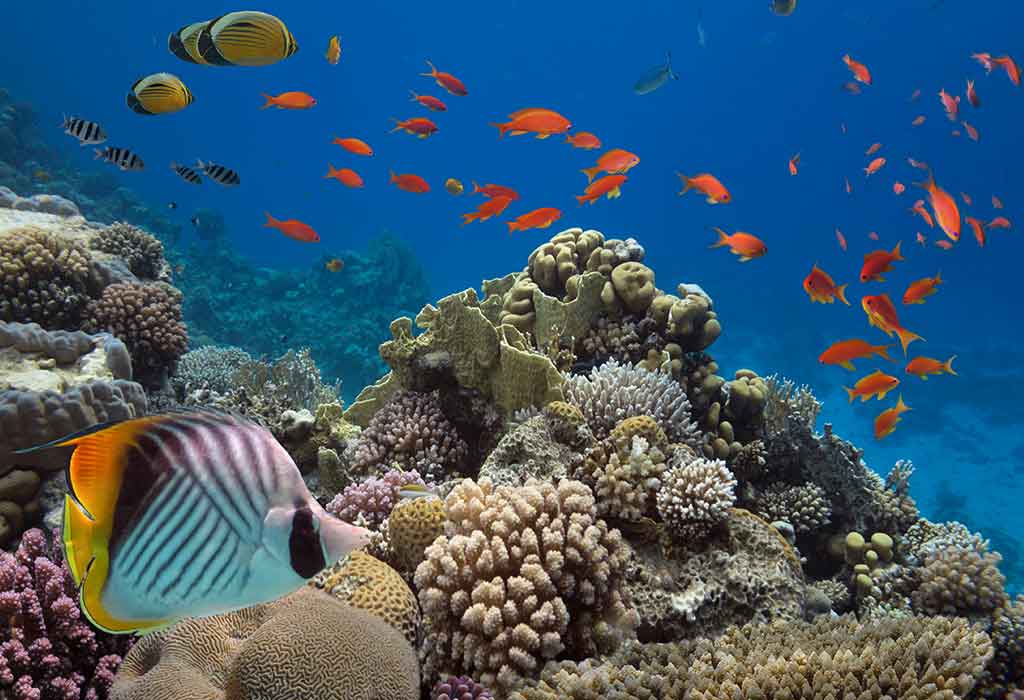This vibrant underwater image captures the rich biodiversity of a coral reef. On the left-hand side, a striking butterflyfish takes prominence, boasting a vivid yellow-orange tail, aqua-colored body adorned with purplish stripes, and a thick white band crossing its eye and face. Surrounding this colorful fish, the reef showcases an array of corals including brain coral in the foreground and crenelated corals in the background, adding to the textural diversity. The corals boast shades of cream, pale blue, and pale purple, contrasting beautifully against the impossibly blue oceanic background.

Adding to the scene's dynamism, a school of around 30 bright orange fish swim on the right side, reminiscent of goldfish in hue. Above them on the left, four black and white striped convict fish and three yellow fish are visible, creating a lively tableau of aquatic life. The corals form an intricate underwater landscape with shapes resembling sponges and peaks of varied textures and colors, from tan to off-white to brown.

In essence, this underwater photo is a mesmerizing snapshot of marine life, teeming with vividly colored fish and the complex, living architecture of corals bathed in a crystalline blue sea.